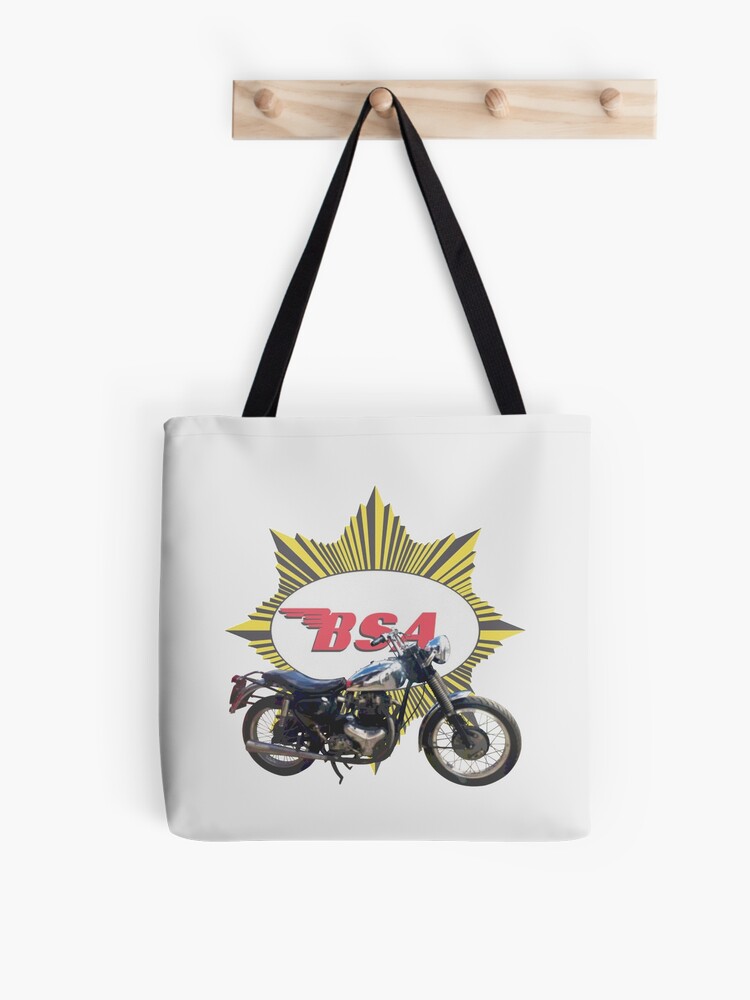The image showcases a light beige, off-white tote bag adorned with a realistic-looking motorcycle and B.S.A. in red letters. Surrounding the B.S.A. text is a star-like symbol, made up of black and gold lines, adding a vintage flair. The tote bag, which is empty, hangs from the second peg of a light tan, brown wooden pegboard mounted on a white wall. The pegboard has four small pegs reminiscent of coat hangers. The bag features a black strap, and the lighting in the image creates a subtle shadow on the left side of the tote. This clean, simple, and advertisement-like photograph emphasizes the tote bag and its detailed design without any additional colors or text, bringing attention solely to the bag and the pegboard against the minimalist backdrop.